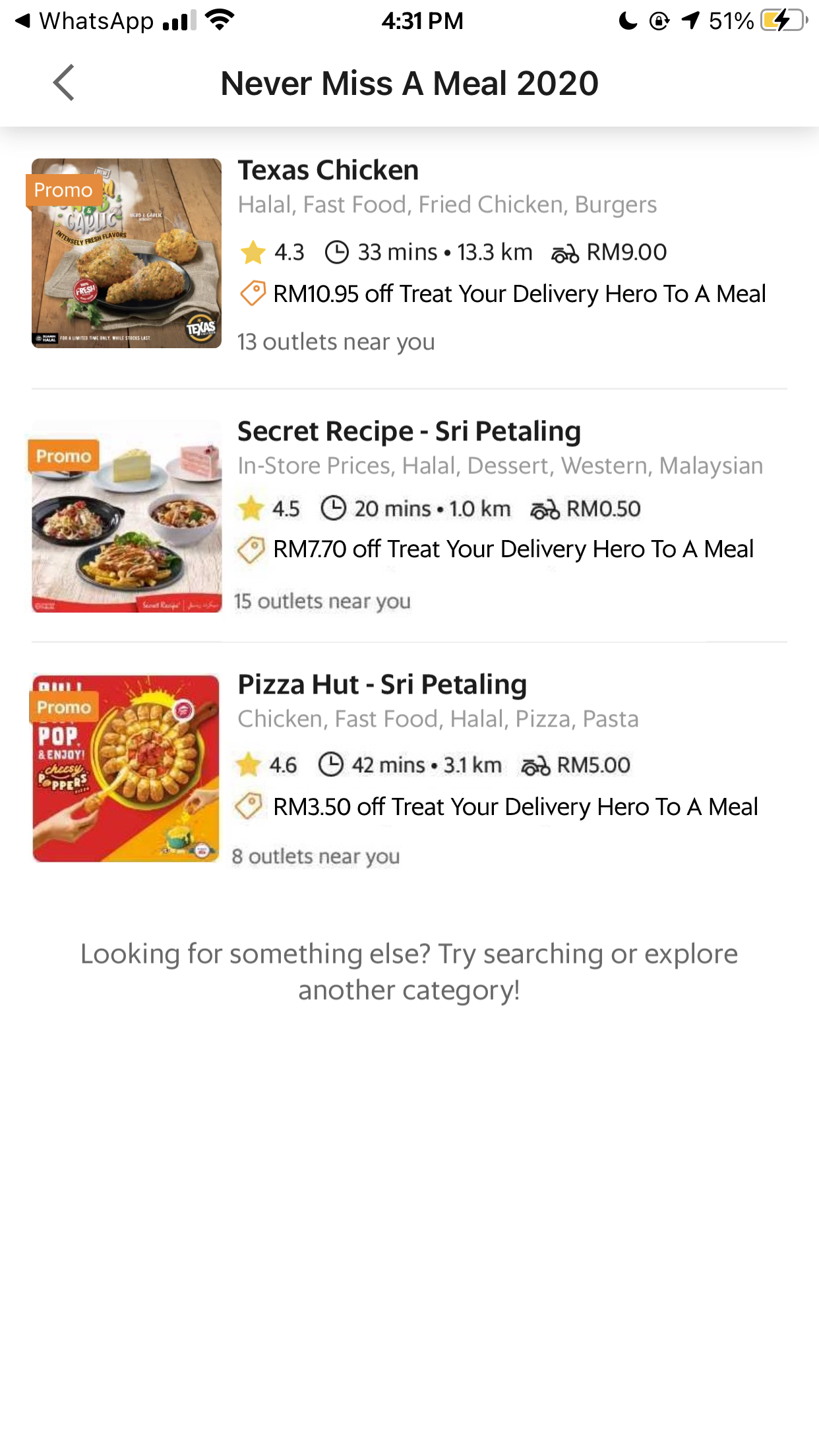The screenshot displays a phone interface, predominantly featuring a list of food delivery advertisements. At the top left corner, there's a back arrow labeled "WhatsApp". The notification bar shows three out of four signal bars, a Wi-Fi icon, the time as 4:31 p.m., a crescent moon icon indicating rotation lock is enabled, and the battery level at 51%.

In the middle of the screen, the header reads "Never miss a meal 2020". Below the header, there is a sequence of food advertisements:

1. **Texas Chicken**:
   - Image: On the left, a photo of fried chicken with a promo tag.
   - Details: "Halal fast-food, fried chicken, burgers. Rated 4.3 stars, estimated delivery time 33 minutes, 13.3 kilometers away, priced at RM 9.00."
   - Promo Code: "Treat your delivery hero to a meal"
   - Availability: "13 outlets near you"

2. **Secret Recipe Sri Petaling**:
   - Image: On the left, a photo featuring bowls of food.
   - Details: "Promo, in-store prices, halal, dessert, Western, Malaysian cuisine. Rated 4.5 stars, estimated delivery time 20 minutes, 1 kilometer away."
   - Promo Code: "Treat your delivery hero to a meal"

3. **Pizza Hut Sri Petaling**:
   - Image: On the left, a photo of food items.
   - Details: "Promo, chicken, fast-food, halal, pizza, pasta. Rated 4.6 stars, estimated delivery time 42 minutes, 3.1 kilometers away."
   - Promo Code: "Treat your delivery hero to a meal"
   - Availability: "8 outlets near you"

At the bottom of the screen, it prompts: "Looking for something else? Try searching or explore another category."